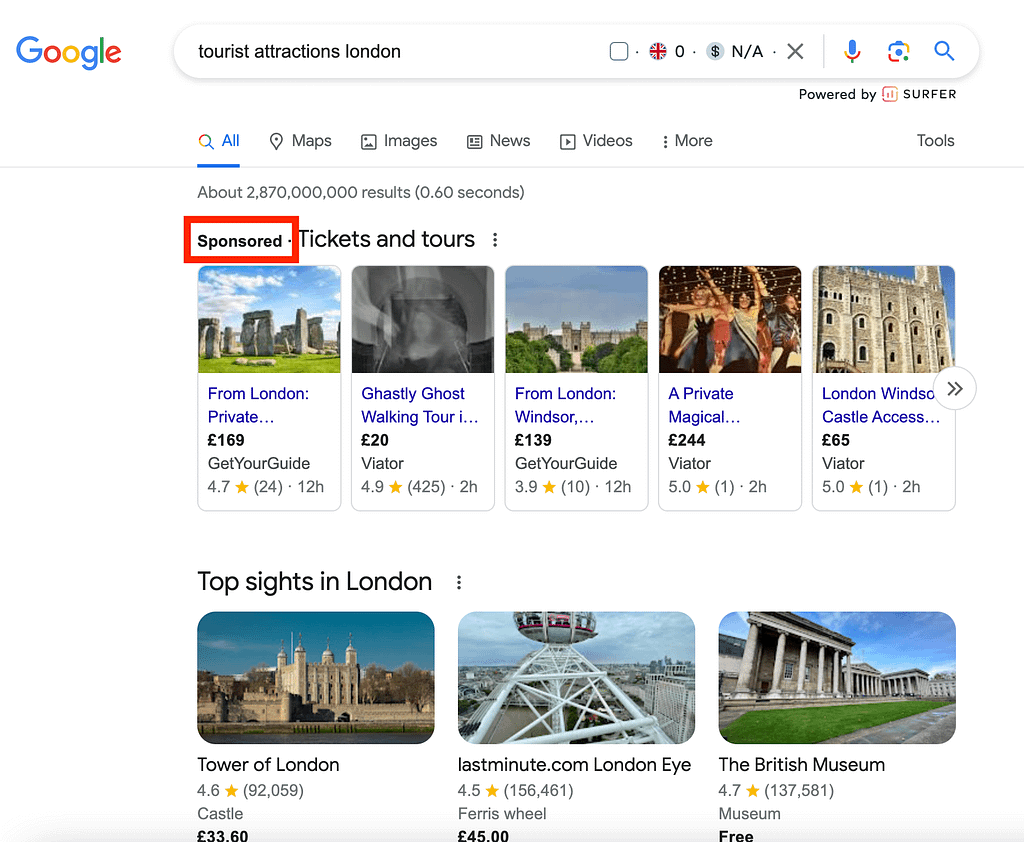**Screenshot of Google Search Results for "Tourist Attractions London"**

In the screenshot, a Google search engine results page is displayed. The search query "Tourist Attractions London" is entered in the search bar positioned next to the Google logo. Within the search bar, there are icons for a British flag, a microphone, an image, and a magnifying glass. The page is powered by Surfer.

Below the search bar, navigation tabs labeled "All," "Maps," "Images," "News," "Videos," and "More" are present, with "All" underlined to indicate the selected option. The "Tools" button is also below these tabs. The search results indicate there are approximately 2,870,000 results found in 60 seconds.

A sponsored section is highlighted by a red bar and displays several tourist attractions alongside their associated images and details. This section includes:

- **Stonehenge:** From London, Private Tour, £169
- **Ghastly Ghost Walking Tour:** £20
- **Windsor Castle:** Entry, £139
- **Private Magical Tour:** £244 (incomplete description)
- **Tower of London:** £3360
- **London Eye:** £45
- **British Museum:** Free

Each entry provides a combination of pricing, tour types, and attraction names to offer a variety of options for tourists visiting London.